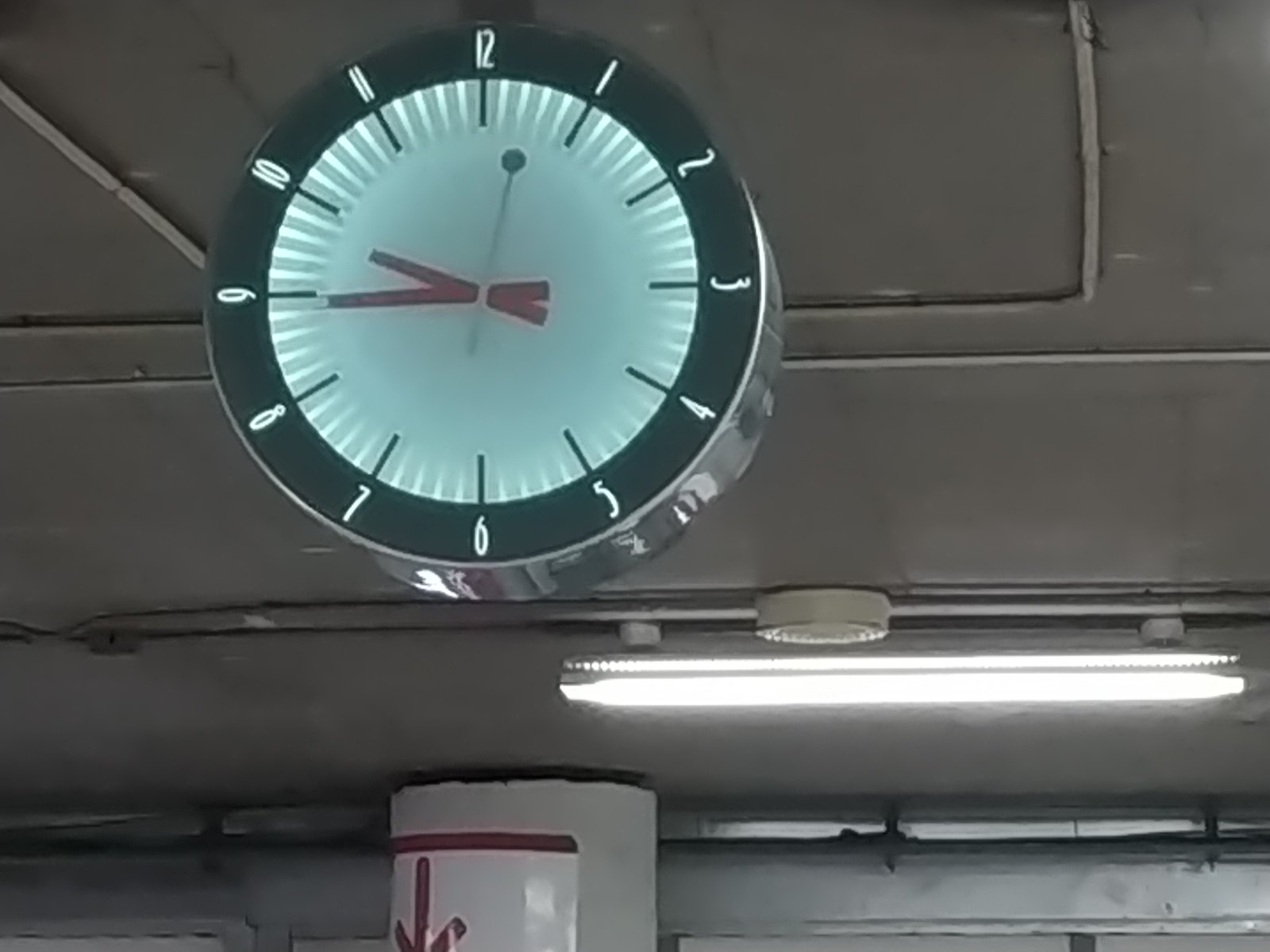This photograph depicts a prominently lit industrial-style clock, likely crafted from stainless steel or a similar metallic material. The frame of the clock is black, contrasting sharply with its illuminated white face, and features clearly visible numbers from 12 through 11 in a bright digital display. The clock's hands add a striking visual element: the hour and minute hands are painted red, while the second hand is white with a distinctive black dot at its tip. Black numerals mark the hours, complemented by white minute markings, ensuring high visibility against the luminous face. 

The clock is mounted on a grayish ceiling, suggesting a utilitarian or industrial environment. In the background, a long, white light fixture adds to the atmosphere, casting even illumination across the scene. A notable feature within the space is a post with a downward-pointing red arrow, hinting at directional guidance. This setting might resemble a garage, an outdoor structural facility, or possibly a subway train station, though the exact location remains ambiguous. The elements combine to evoke a functional, yet somewhat mysterious, urban backdrop.